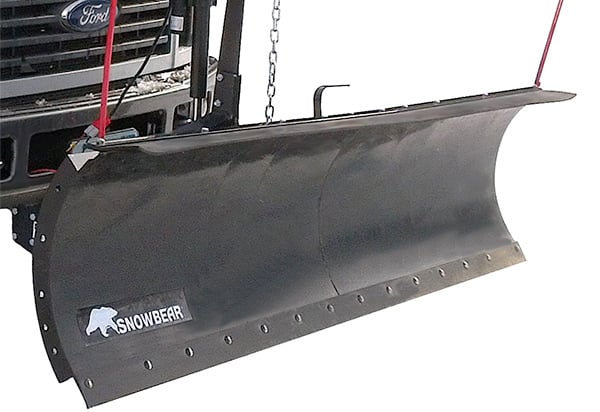This close-up image features a heavy-duty SnowBear snow plow attached to the front of a Ford truck, which is partially visible in the top left corner. The Ford truck is identifiable by its navy blue oval logo with the cursive "Ford" emblem on the grill. The snow plow is black and made of metal, with a slightly curved blade designed for efficient snow pushing. The SnowBear logo, located at the bottom left corner of the plow’s blade, features white lettering and an outline of a polar bear against a black background. The plow is held up by a red strap on both ends and a silver chain that connects more towards the center, further secured by thicker black bars. The background of the image is entirely white, highlighting the plow and truck without any additional scenery, suggesting that the focus is on showcasing the snow plow, potentially for advertising purposes.